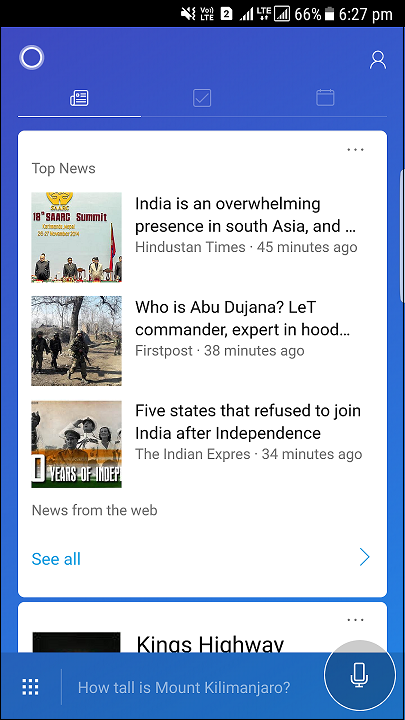This image is a screenshot taken on a cellular device displaying a news application interface. The phone has full carrier signal strength on an LTE network, with a battery life at 66%. The screenshot was captured at 6:27 p.m. The interface features a blue background, with a prominent white circle at the top, outlined by another circle. To the right of these circles, there's a profile icon depicting a head and shoulders silhouette. 

At the very top of the screen, a white icon representing a phone and fax is highlighted, indicating it has been selected. Below this, the app presents top news stories. The first article is titled "India’s Overwhelming Presence in South Asia" from the Hindustan Times, posted 45 minutes prior. This article includes a photograph showing three men seated at what appears to be a press table. Below it, there is another article with the headline "Who is Abu Dajjana, Lead Commander." 

Additionally, an alarm notification symbol with an 'X' through it is visible, indicating that notifications are possibly muted or dismissed.